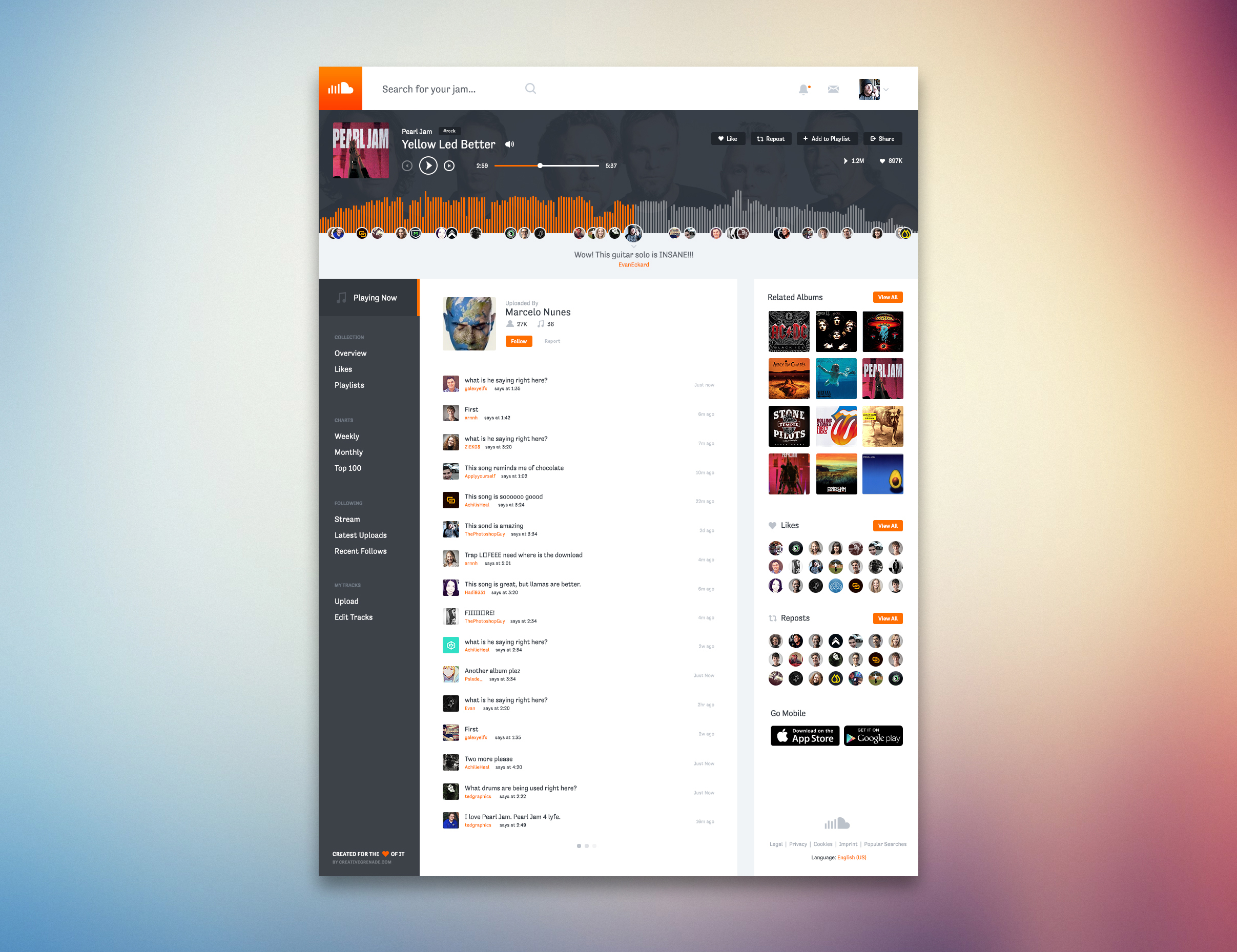The image is a vibrant and colorful webpage dedicated to the iconic band, Pearl Jam. At the very top of the page, there is a prominent black strip housing the search bar, where "Pearl Jam" has been entered. Below the black strip, a bar graph features orange on the left side gradually transitioning to gray. This interface allows users to click a button to play one of Pearl Jam's songs, currently shown as halfway played.

On the left, the band's name, "Pearl Jam," is displayed in striking white text above a pink image. Above this, a small image of a man's head signifies the currently playing track. As you move down the page, a comprehensive list of songs by Pearl Jam is detailed.

A dark gray box occupies the left side of the screen, while a column on the right showcases all the album covers from Pearl Jam's discography. Beneath these album covers, additional songs are listed, providing options to purchase them through Apple Music or Google. The overall design of the webpage is both functional and visually engaging, celebrating the music and legacy of Pearl Jam.